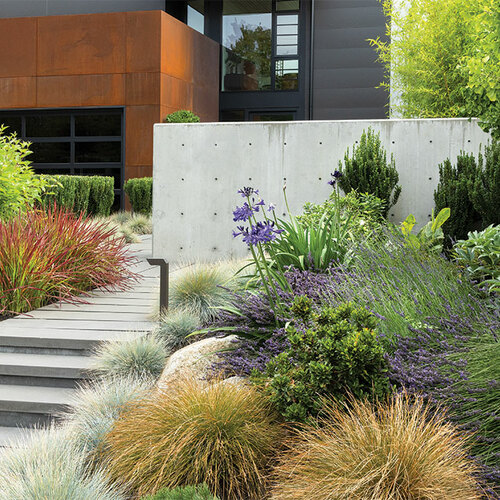The photograph captures an outdoor scene during daytime with natural light, focusing on the walkway leading up to a modern, cubical-designed house. The walkway, starting from the bottom left corner, is composed of gray wooden planks and includes three steps on the left side, which lead around a low gray concrete wall. The house is rectangular with a blocky, architectural design. The lower section is a dark brownish-orange color featuring a rolling garage door, while the upper section is dark gray, adorned with large, single-pane windows in black frames.

The landscaping around the walkway is meticulously curated, featuring a variety of plants. On either side of the walkway, the vibrant garden includes round-shaped white and green plants, yellow and green foliage, as well as purple flowers and red and green plants. Square-shaped bushes adorn the area around the building, enhancing the modern aesthetic. A tree is visible in the upper right corner, adding to the lush surroundings. The thoughtful and diverse plant arrangements showcase extensive landscaping efforts, contributing to the overall sophisticated and elegant appearance of the property.